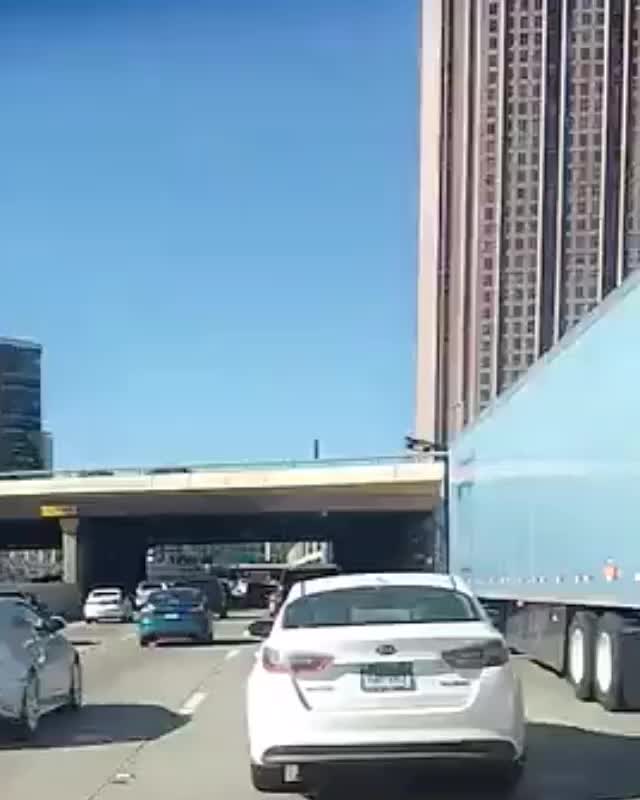In this bright, cloudless daytime scene, we observe a bustling city interstate featuring four lanes filled with a mix of cars and trucks. Directly ahead is a white Kia sedan, positioned adjacent to a sizeable tractor-trailer truck that appears bluish, likely reflecting the sunlight which gives it a silvery tint. Ahead looms a bridge spanning the width of the interstate, while to the right, a towering skyscraper rises, forming part of the city's skyline. The clear light blue sky enhances the vivid shadows cast by the vehicles, including a noticeable shadow of another car on the road. The urban landscape captured conveys the dynamic energy of city traffic under a pristine, azure sky.